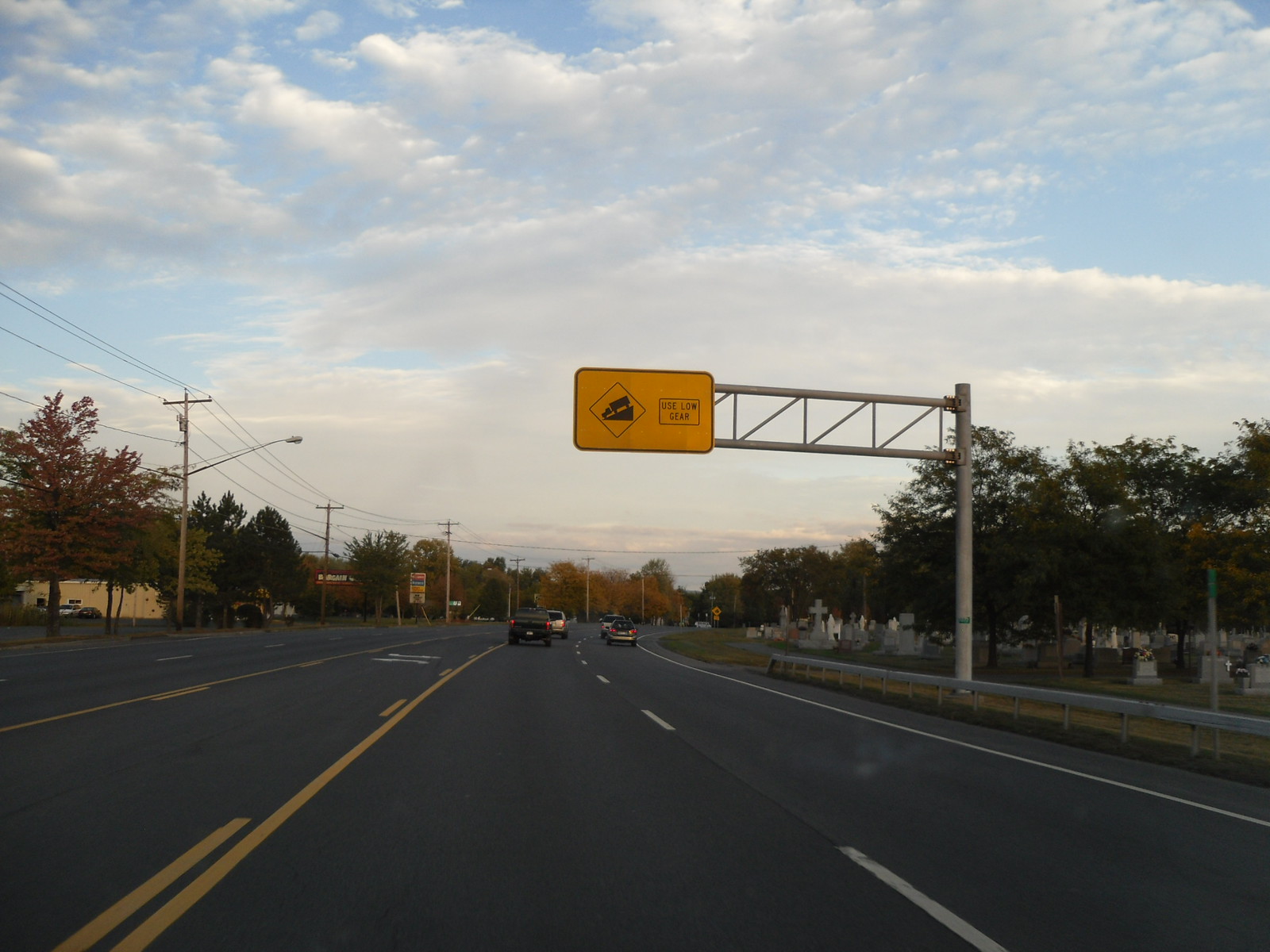This photograph captures a serene yet slightly ominous scene taken from a highway. The image appears to be shot from a perspective in the middle of the road or perhaps from a moving vehicle. Ahead, a few cars are seen driving away, their destination unknown as they head down the two-lane highway, which is separated by a slender median. 

Flanking the road, a dense arrangement of trees offers a natural border, while to the left, business signs emerge in the distance alongside a scattering of buildings. Telephone lines run parallel to the highway, adding a touch of connectivity to the otherwise isolated stretch of road. On the right side, an expansive cemetery stretches out, dotted with approximately a hundred headstones, quietly marking the area and introducing a contemplative atmosphere. 

Closer to the viewpoint, a metal railing runs along the roadside, next to a prominent yellow sign jutting out towards the road, likely indicating an upcoming height restriction—perhaps hinting at an approaching bridge. The scene is bathed in midday light, with soft cumulus clouds punctuating the sky against a backdrop that suggests a calm yet potentially rainy late afternoon. The sun peers through the clouds intermittently, casting gentle shadows and highlighting the varied textures within this multifaceted landscape.